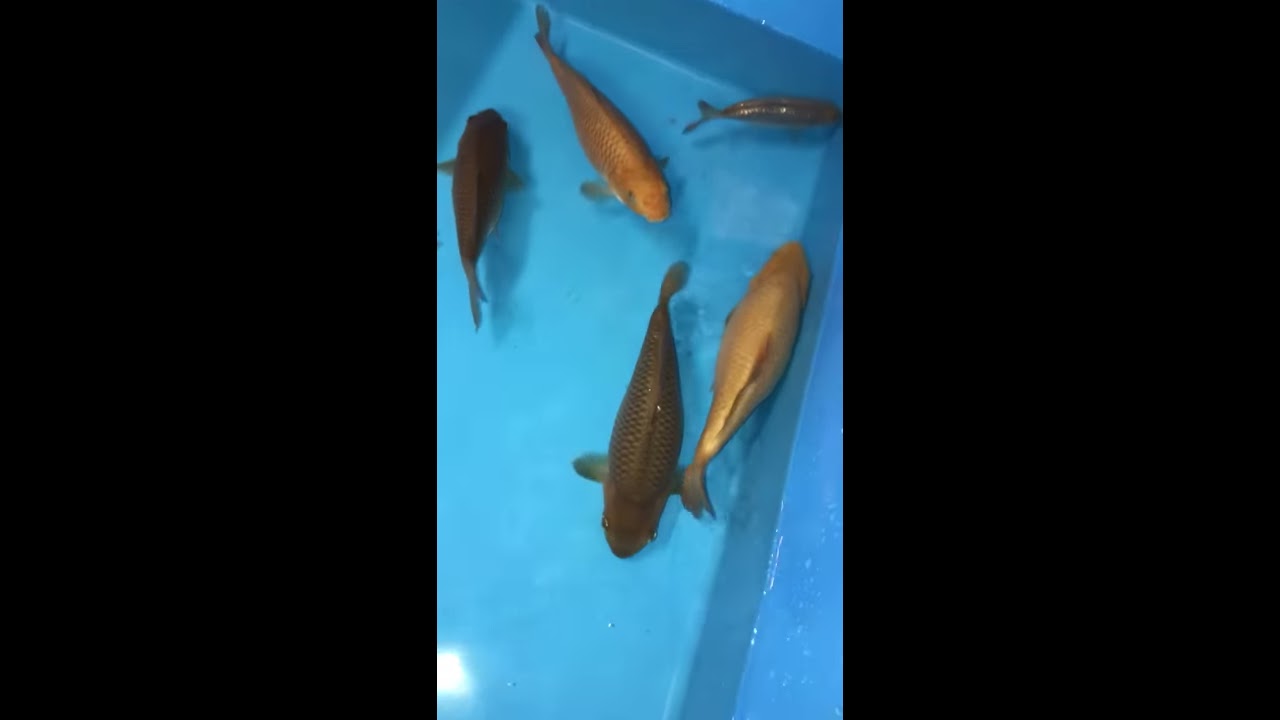The image depicts a scene with three vertical rectangles, where the left and right rectangles are black, framing the central image. In the middle rectangle, there is a light blue rectangular basin filled with water, reminiscent of a fish market container. Within the basin, five fish can be seen. On the right side, the two largest fish are positioned; one has a lighter color and faces upwards, pressed against the side of the basin, while the other, darker fish faces downwards. The top right corner houses a smaller, gray fish facing into the corner. On the top left, another fish's tail points towards the corner, with its face angling downward toward the bigger fish on the right. Additionally, on the bottom left of the image, there is a reflection of white light. The setting suggests an illuminated scene, possibly taken from a cell phone, giving it a social media feel, such as a TikTok video. The overall container and setting give the impression of a market environment but no humans other than the potential camera holder are visible.